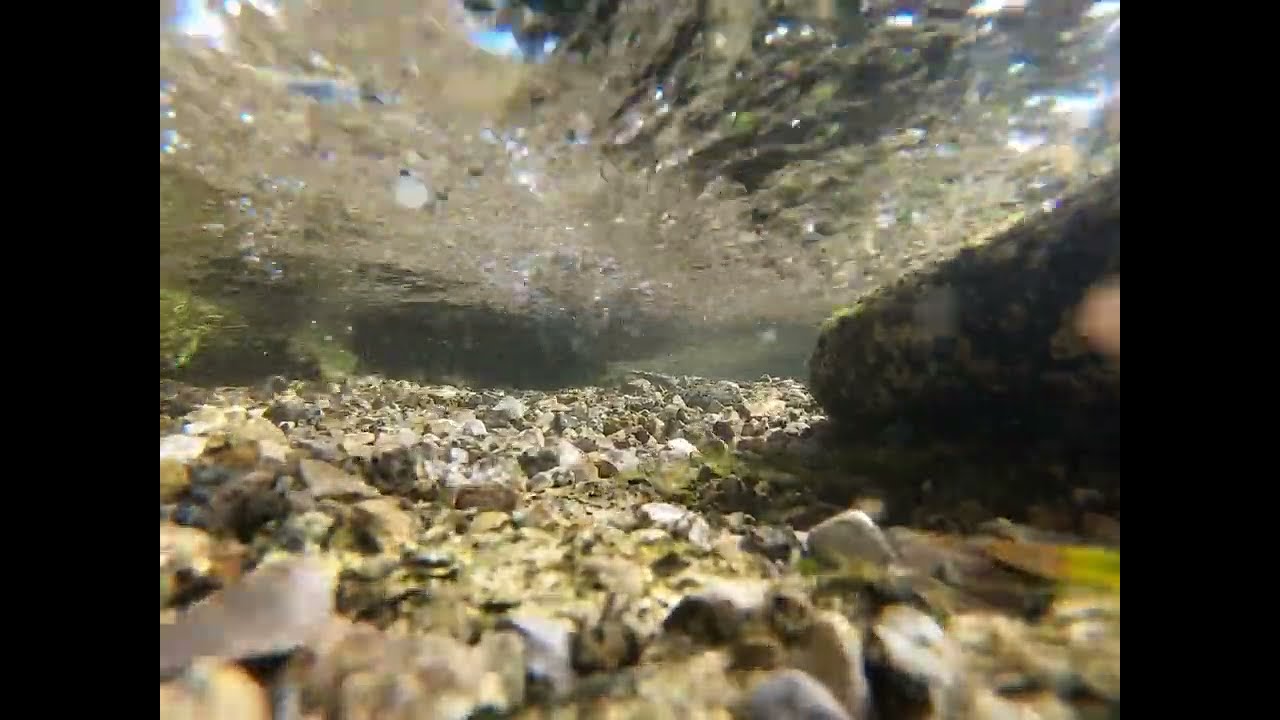The photograph captures the serene underwater landscape of a shallow lake on a clear day. At the top of the image, the water's surface can be seen, rippling slightly beneath beams of blue sky. The clarity of the water reveals a diverse collection of rocks in various hues—gray, white, brown, tan, black, greenish, and orange—scattered across the lakebed. Dominating the right side of the frame is a substantial rock formation, with an even larger formation on the left, occupying nearly half of the picture. Among the rocks, patches of green seaweed and grasses are visible, adding texture and color to the scene. The blurred background hints at tall green and brown trees lining the lake's shore, with glimpses of the sky piercing through, reinforcing the tranquil, daylight setting.